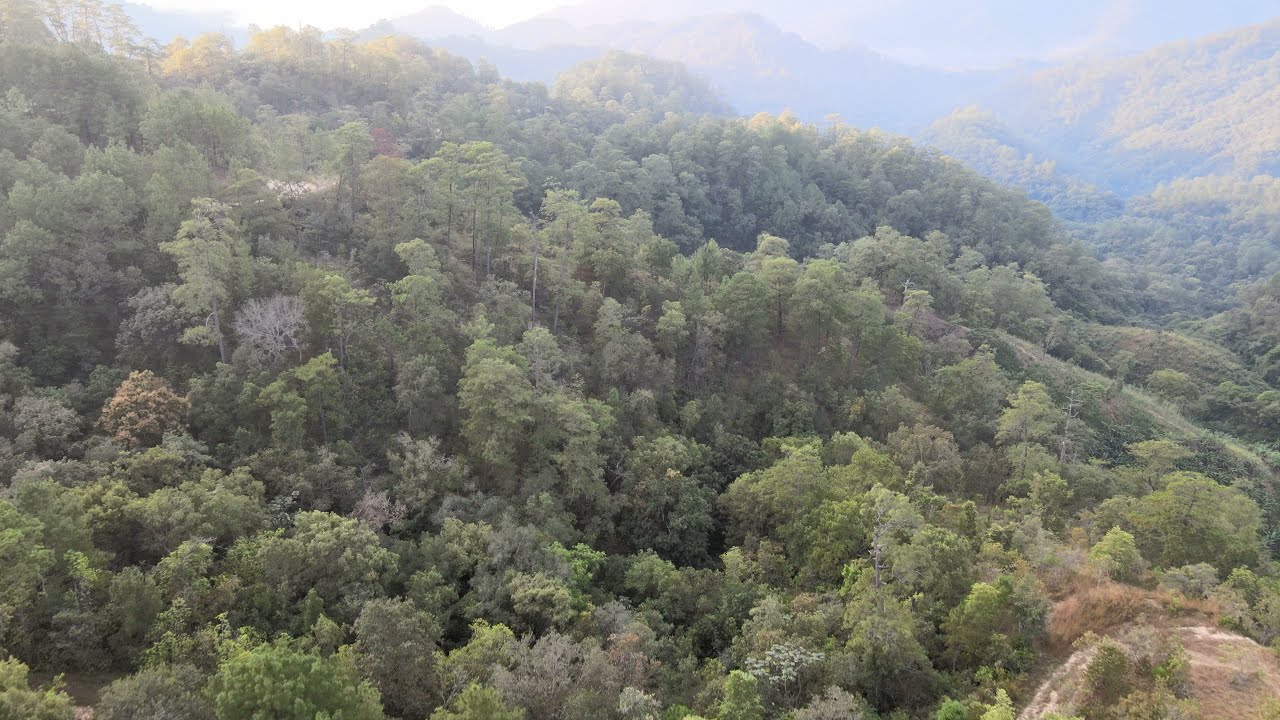This captivating photo showcases a lush mountain scene, dominated by an expansive, dense forest of trees in varying shapes and hues. The vibrant greenery, ranging from dark green to lighter shades and even some yellowish tones, suggests the season is spring or summer. In the foreground, there are smaller hills and peaks, interspersed with patches of dirt and hints of trails, possibly indicating areas where people might traverse. The image offers a layered perspective, with a slight downward angle giving an overhead view of the tree-covered landscape. As your gaze moves toward the background, you see distant mountains gradually fading into a misty horizon, lending a sense of depth and majesty to the scene. A small strip of sky is visible in the upper left corner, enhancing the serene, natural beauty of this mountain panorama.